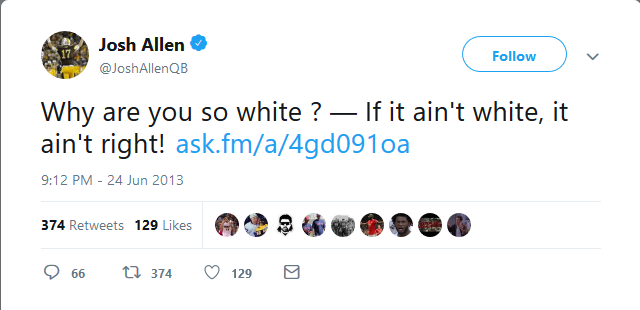This is a screenshot of a Twitter post featuring a single tweet dated June 24th, 2013, at 9:12 PM. The image is from the Twitter light theme, evident from the tweet's white background. The username and avatar of the tweeter are visible in the upper left corner. The avatar is a circular image depicting a football player with his back to the camera, wearing a crimson jersey with the number 17, a white helmet, and possibly yellow pants. The name "Josh Allen" appears next to the avatar, accompanied by a blue verified icon.

Josh Allen's Twitter handle, @JoshAllenQB, is displayed below his name. In the upper right corner of the tweet, there is a follow icon followed by a small downward arrow indicating a dropdown menu. 

The main body of the tweet reads: "Why are you so white? - If it ain't white, it ain't right!" A URL, highlighted in blue, follows the text. At the bottom of the tweet, engagement statistics are shown: 374 retweets, 129 likes, and 66 replies.